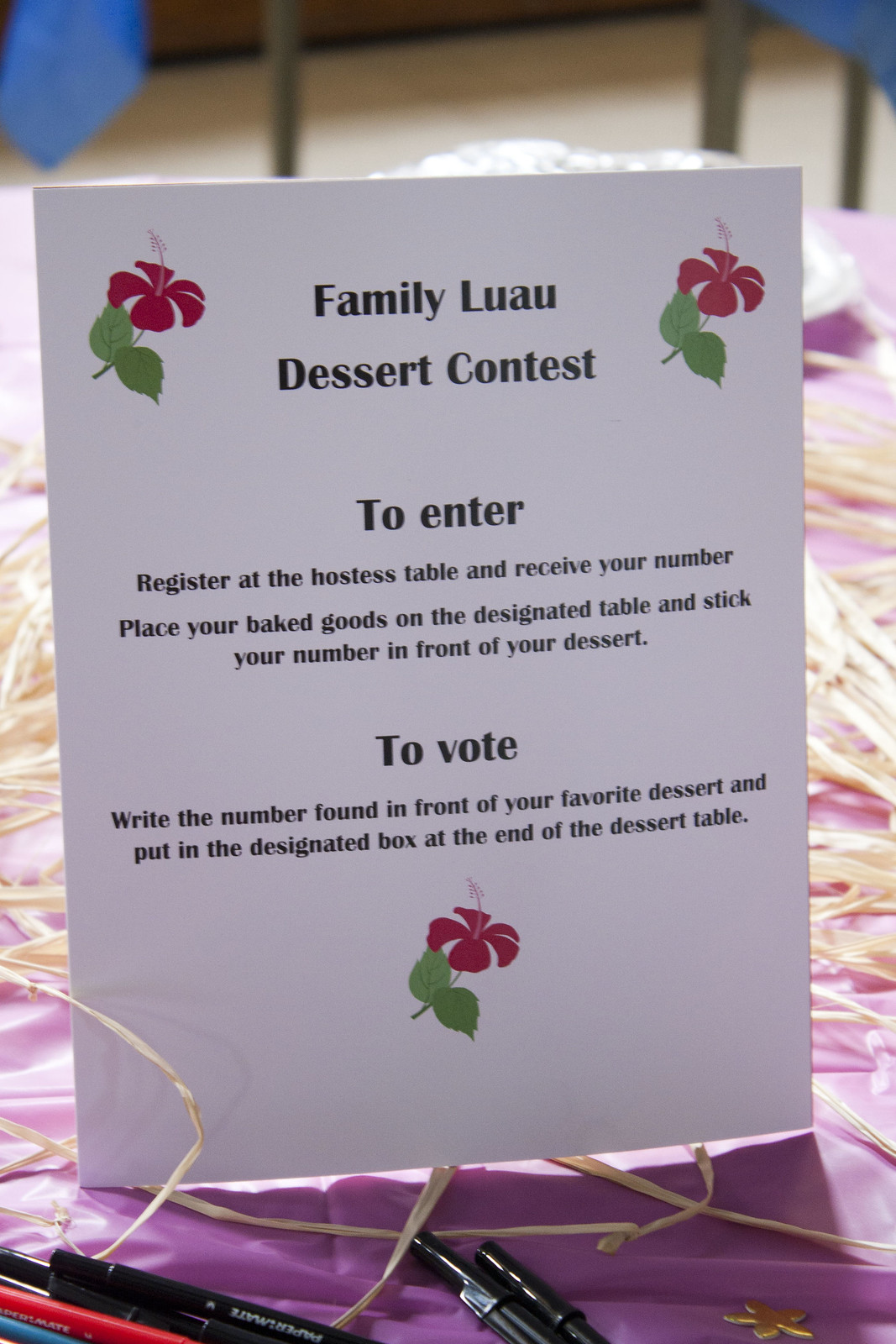The image showcases a white placard positioned on a table with a pinkish-purple orchid-colored fabric, appropriate for a luau-themed event. The placard, which is lit from behind casting shadows forward, prominently displays the title "Family Luau Dessert Contest" in black text. Instructions follow beneath the heading, detailing the process for entering and voting in the contest: to register at the hostess table, receive a number, place baked goods on the designated table with the number affixed in front, and write the number of your favorite dessert to submit into a designated box for voting. The decoration includes three vibrant Hawaiian flowers; two pink with green leaves in the top left and right corners, and one centrally placed at the bottom of the placard. Scattered on the table, in addition to the floral-themed elements, are some strips of raffia or dried grass, pens, and papers. In the distant background, the wooden floor is visible, reinforcing the interior setting of the event.